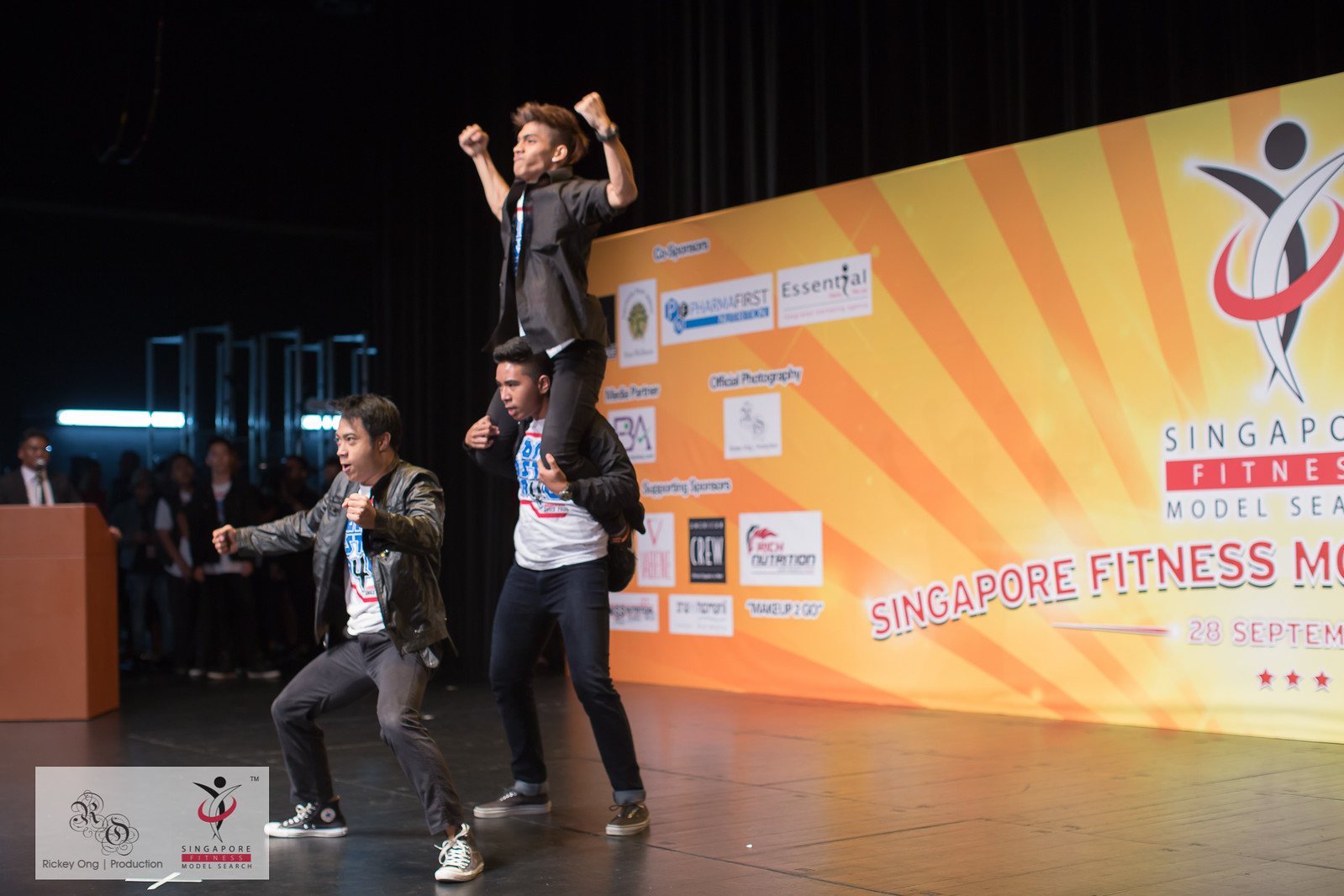In this full-color indoor photograph, we see three men striking a dynamic pose on a black stage, likely at a fitness competition titled "Singapore Fitness Model Search," based on a partially visible yellow banner in the background. The man in the front is adopting a squatting stance, dressed in black jeans, a black jacket, and a white t-shirt, with his arms extended in front of him in fists. Behind him, another man, similarly dressed in a black jacket and dark blue jeans, is holding a third man on his shoulders. This man on top is wearing a short-sleeved black shirt and black pants, flexing his muscles with his arms raised and his face showing determination. To the left of the stage, there are a few more people visible, one of whom stands at a dark brown podium, possibly addressing the event. In the bottom left corner of the stage floor, there is a white watermark accompanied by two additional logos.